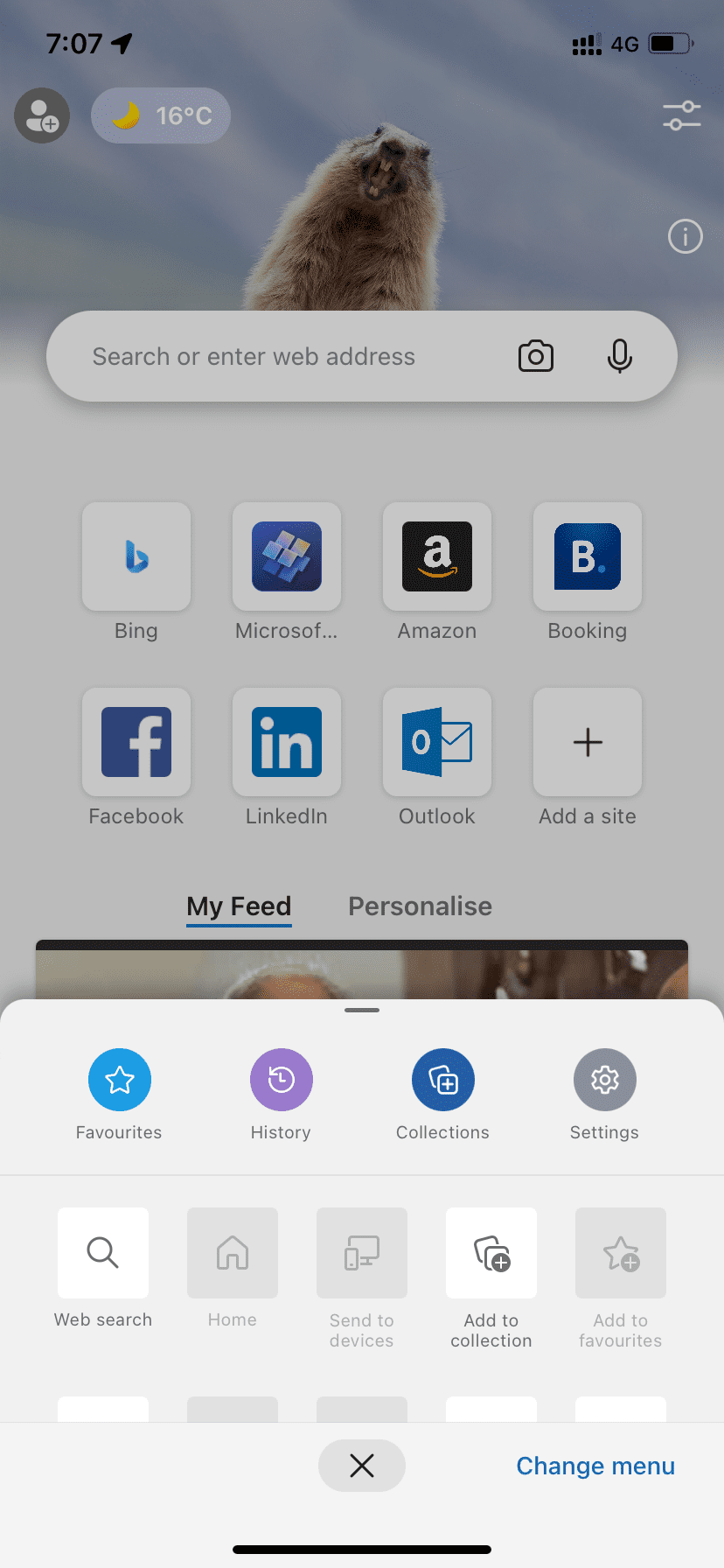This image is a detailed screenshot of a smartphone's home screen. 

At the very top, the status bar displays the current time on the left and indicators for Wi-Fi connectivity, 4G signal, and battery life on the right. Below the status bar on the left, there is a circular icon depicting a head and shoulders, and beside it, another circular icon showing the current moon phase and a temperature reading of 16 degrees Celsius.

Above the main content, a playful image of a beaver peeks over the top of a search bar, giving the impression that the beaver is looking directly at the user. Below the search bar are two rows of app icons: the first row includes Bing, Microsoft, Amazon, and Booking; the second row features Facebook, LinkedIn, Outlook, and an option to "Add a Site."

Further down, there are sections labeled "My Feed" and "Personalize." Just below these, a partially visible second image can be seen, which appears cut off due to an upward swipe. This reveals additional options including "Favorites," "Histories," "Collections," and "Settings," which span across the top of a swipe-up bar. The bar also contains shortcuts for "Camera Control Center," "Web Search," "Home," "Center of Devices," "Add to Collections," and "Add to Favorites."

At the bottom of the screen, a prominent "X" symbol is visible along with the option to "Change Menu." 

Overall, this screenshot provides a comprehensive view of the user's organized and personalized smartphone home screen interface.